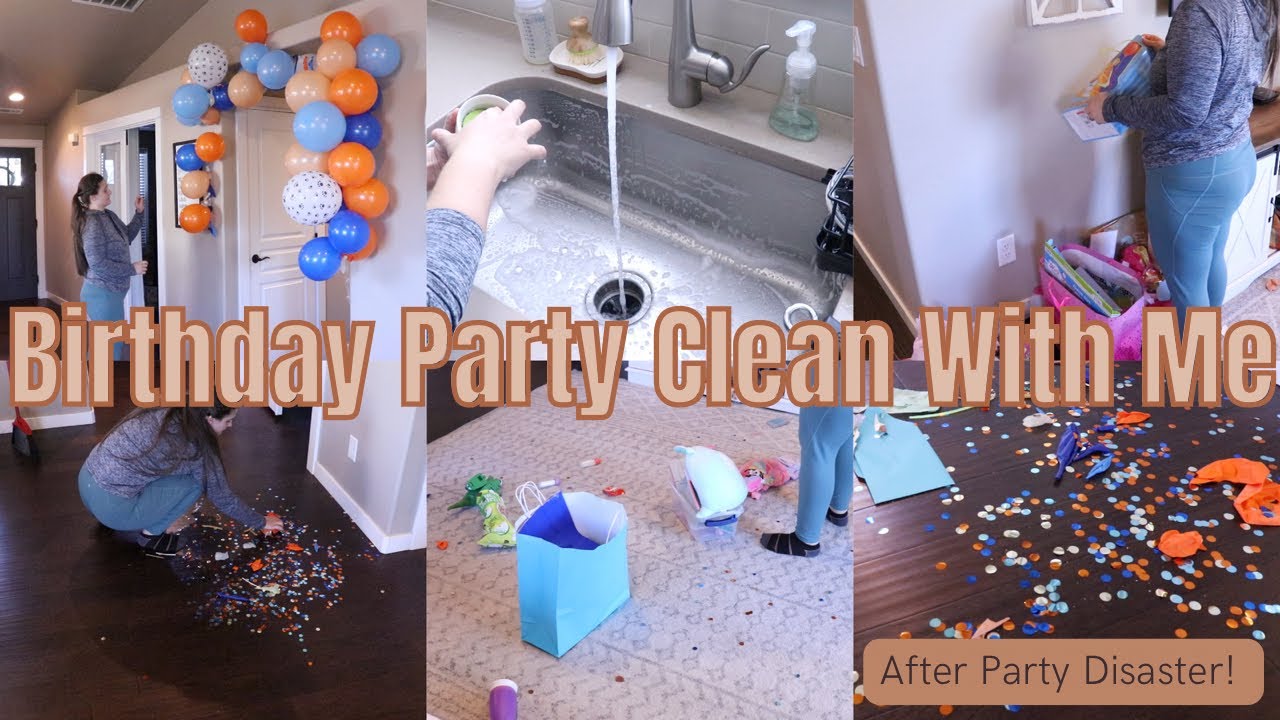The image is composed of three vertically aligned panels with the central text "Birthday Party Clean With Me," displayed in a light pink font with a darker pink outline. The first panel on the left shows two women, one standing and one crouching, setting up for a party. They are surrounded by scattered items, possibly uninflated balloons, and there is a colorful balloon arch around a doorway. The middle panel features two sub-images: the upper section depicts hands washing dishes in a stainless steel sink with water running, presumably cleaning up after the party. The lower section shows random items, including a blue paper bag, on the floor with someone in blue leggings and stocking feet standing over them, seemingly organizing or picking up. The right panel is also divided into two sub-images, accompanied by the text "After Party Disaster" with an exclamation mark. The upper image shows the same individual in blue leggings folding items, while the lower sub-image focuses on a floor littered with broken balloons, multi-colored confetti, and assorted party debris, which the person appears to be cleaning and placing into a trash container.